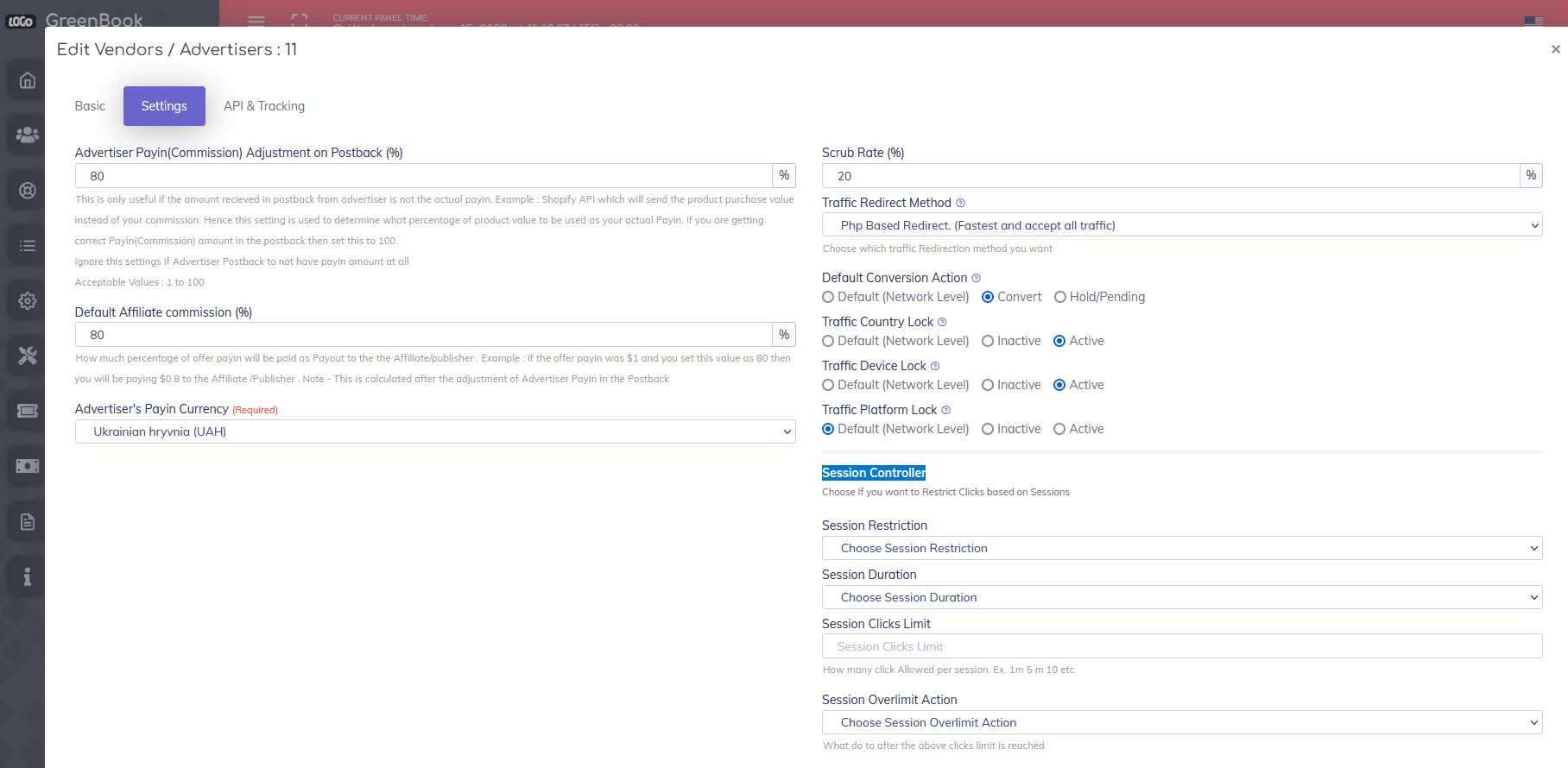This is a detailed screenshot of a web interface featuring a large pop-up menu that occupies most of the screen, partly obscuring the main website. The background of the main site is gray, visible only as thin slivers along the top and left edges of the screen.

The pop-up menu, positioned in the upper left corner, has a white background and dominates the view. At the very top, the menu is titled "Edit Vendors/Advertisers: 11," displayed in black font. In the upper right corner of the pop-up, there is a small "X" icon for closing the menu.

Directly below the title, there are four clickable options in gray font: Basic, Settings, API, and Tracking. The "Settings" option is currently selected, indicated by a blue highlight that surrounds the word, turning the text white.

Under the "Settings" heading, black text reads "Advertiser Commission Adjustment on Postback," although the text is somewhat blurred and difficult to decipher due to the low image quality. Below this, there is a text field or drop-down menu displaying the number "80." Further down, there is an area filled with unreadable gray text.

Subsequently, another label reads "Default Affiliate Commission Percentage," adjacent to another field also containing the number "80." Below this are two more lines of unreadable gray text. Finally, the menu option "Advertisers Pay-In Currency" is listed, showing the currency as "Ukrainian Hryvnia."